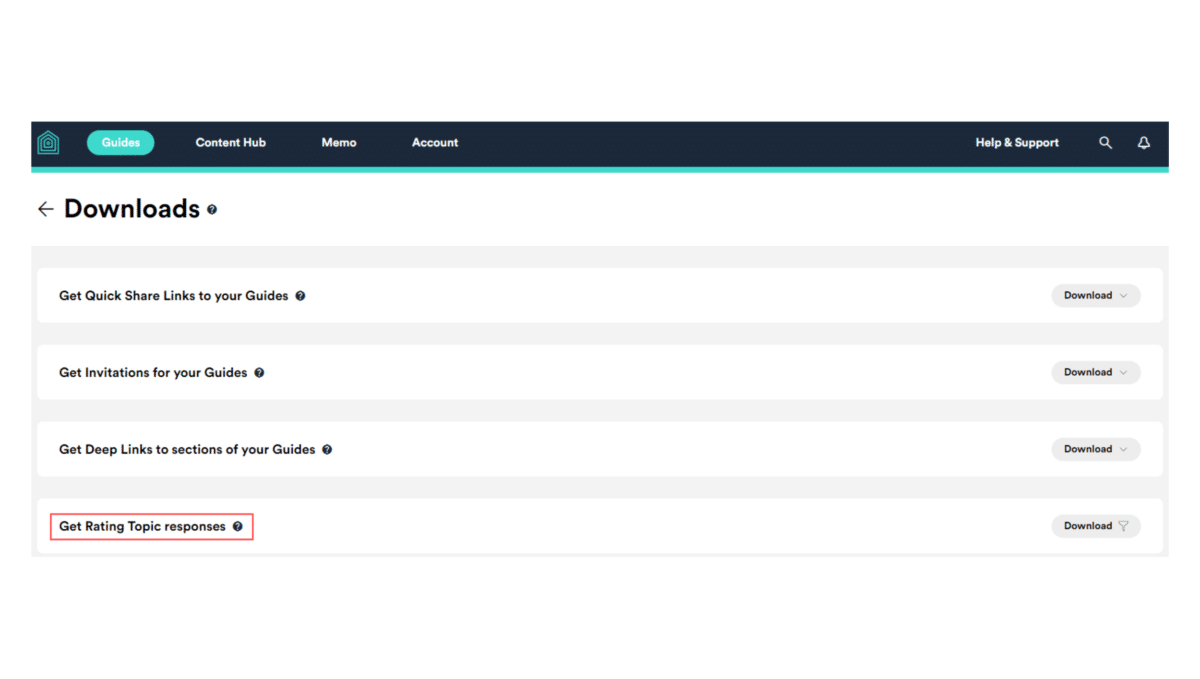This image, taken from a website screen, features a "Downloads" page. At the top, the word "Downloads" is prominently displayed alongside a back button and a circular question mark icon. 

At the very top of the screen, a horizontal black rectangle spans from the left to the right, accentuated with a thin teal-green line running along its bottom edge for emphasis. Within this black header, various icons and text elements are present: a stylized house icon created by continuous lines, followed by the labels "Guides," "Content Hub," "Memo," and "Account." Toward the far right of this header area are icons for "Help and Support," a magnifying glass (presumably for search functionality), and a bell (likely for notifications).

Below the "Downloads" heading, there is a section on the left with various options, each accompanied by a question mark for additional information. These options include:
- "Get quick share links to your guides"
- "Get invitations for your guides"
- "Get deep links to sections of your guides"
- "Get rating topic responses"

The final option, "Get rating topic responses," is highlighted within a red box, suggesting it can be clicked for further action.